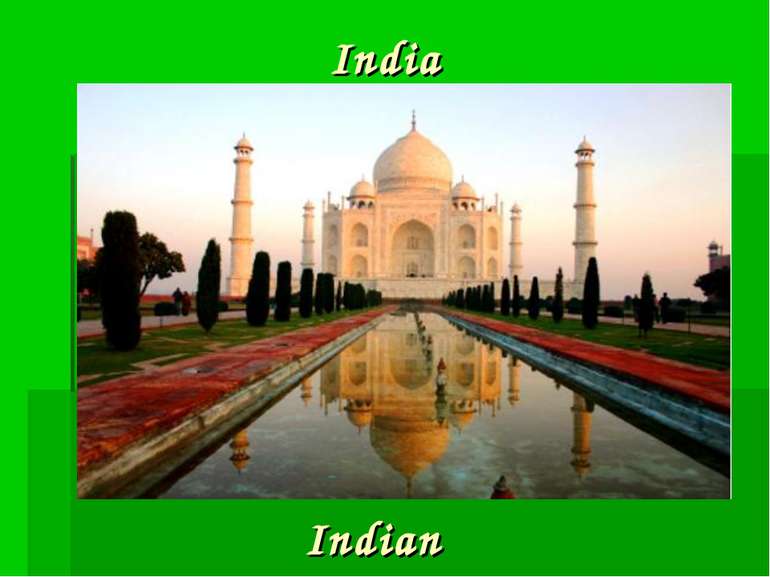This image, rectangular like a PowerPoint slide, features a striking photograph of the Taj Mahal taken from a straight-on perspective as the sun sets. The iconic white marble mausoleum stands prominently against a bright blue sky, with its large central dome flanked by two smaller domes and matching spires on either side. The Taj Mahal's reflection is beautifully captured in the long, narrow reflecting pool directly in front of it. Flanking the pool are well-maintained walkways and symmetrical rows of conical trees and green shrubs, all part of the lush landscaped grounds. In the background, large white pillars add to the grandeur of the scene. The image's backdrop is a gradient green, lighter at the top and darker at the bottom, with additional darker green rectangles adding depth. At the top of the image, the word "India" appears in a white script font, while the bottom reads "Indian" in a matching script font with a cream color and black shadow, framing the visual elegantly. The setting is bright and clear, emphasizing the meticulously symmetrical design and serene beauty of this historic monument, with people visible along the walkways, contributing to the lively yet peaceful atmosphere.